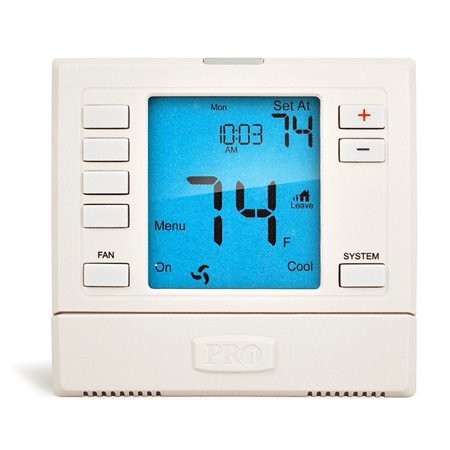**Detailed Description of a Digital Home Thermostat:**

This is a high-resolution indoor close-up photograph of a square, white plastic digital home thermostat. The thermostat features a prominently central blue digital display on the upper two-thirds of its body. The display showcases information in clear black lettering.

Starting from the top, slightly left of the center, the screen displays the day abbreviation "MON." Directly below, it shows the current time, "10:03 AM." To the right of the time, it reads "SET AT" followed by the number "74." Centrally located on the lower half of the display is a larger number "74" with a small "F" beneath the "4," indicating the temperature in Fahrenheit.

On the left side of the display, there are two indicators: one labeled "MENU" and another below it indicating "ON," accompanied by a fan icon. On the lower right side of the display, it reads "COOL."

Surrounding the digital display is a white plastic bezel with an array of buttons. On the left side, there is a vertical column of five rectangular white buttons. Four of these buttons are grouped together at the top without any labels. The fifth button, positioned at the bottom of the column, has the word "FAN" printed above it.

On the right side of the thermostat, there are three similarly shaped rectangular buttons arranged in a vertical column. The top two buttons feature a red plus sign and a minus sign, respectively. Below these, there is a button labeled "SYSTEM."

At the very bottom of the thermostat's front panel, a horizontal line spans the last third of the device, likely indicating the battery compartment. Above this line, there is a raised emblem embossed with the letters "PRO."

This detailed description captures the various features and layout of the digital home thermostat, providing a comprehensive overview of its design and functionality.